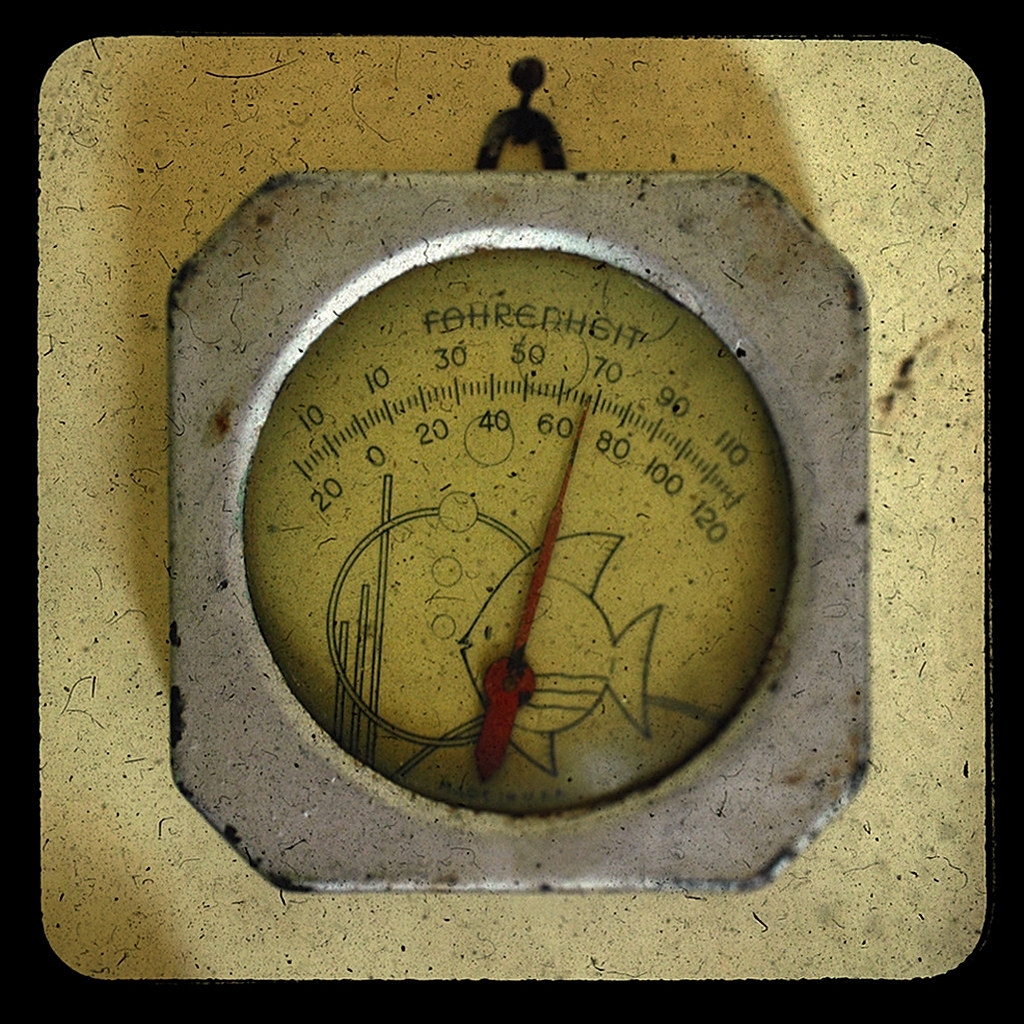This color photograph captures a close-up of an antique temperature gauge mounted on a beige, tile-like plaque. The outer frame of the gauge, resembling pewter with a silvery hue, shows signs of aging with a developed patina at the corners. The round dial features a mustard yellow face, prominently displaying the word "Fahrenheit" at the top. The numerical markings form a semicircle, starting from 10 on the left and increasing in increments of 20 (10, 30, 50, 70, 90, etc.). A red needle points precisely to 70 degrees, indicating room temperature. Adding a whimsical touch, there is a small schematic drawing of a large fish, enhancing the charm of this vintage piece.